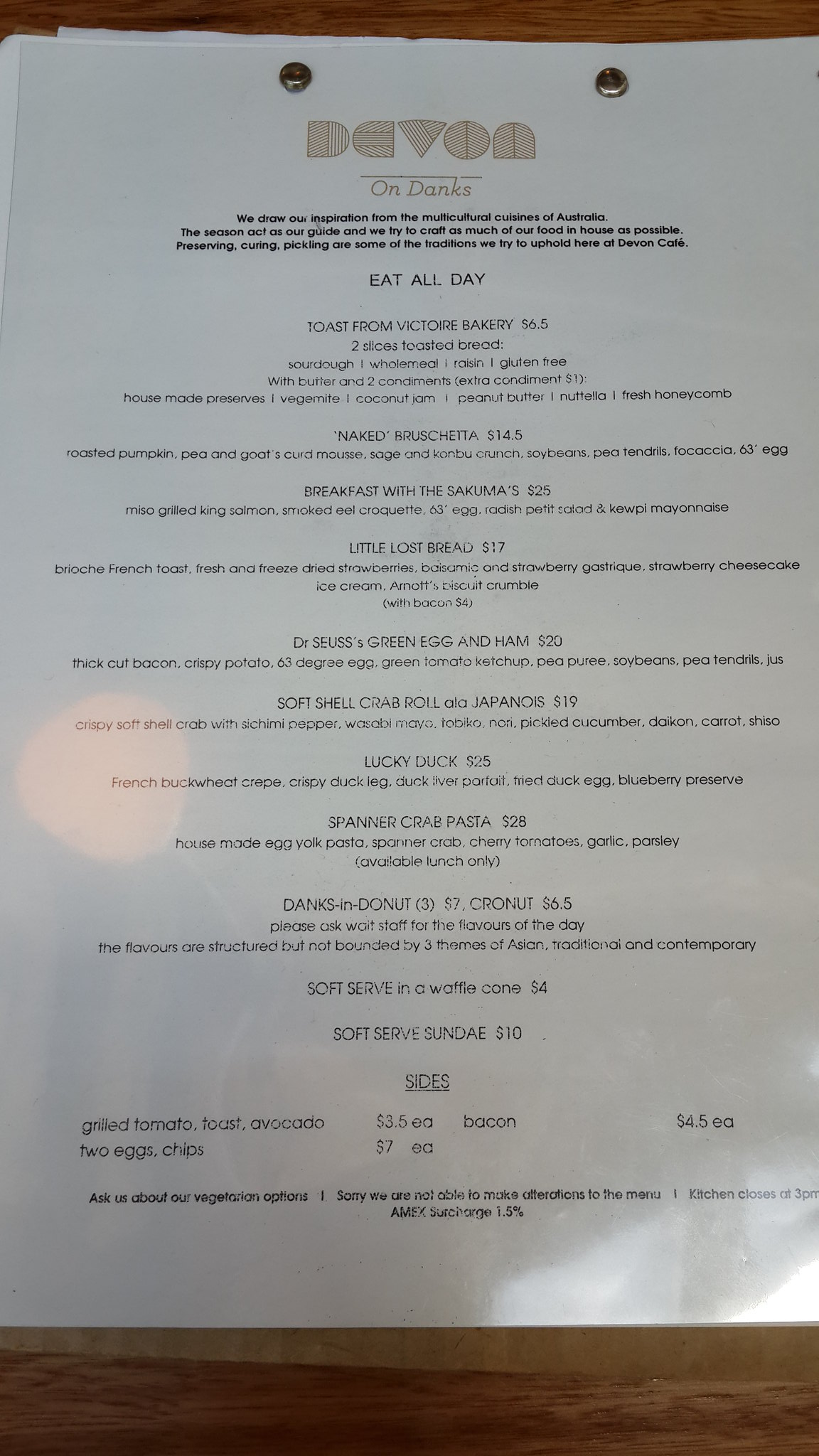This photograph captures a single page from a menu, displayed against a white background with black text. The title "Divan on Donks" is elegantly highlighted in gold script at the top of the page. The section titled "Eat All Day" follows, presenting a diverse selection of dishes described in detail. The offerings include "Toast from Victoire Bakery," "Naked Bruschetta," "Breakfast with Sakuma," "Little Lost Bread," "Dr. Seuss Green Egg and Ham," "Soft Shell Crab Roll," "Lucky Duck," "Spanner Crab Pasta," "Donks in Donut," "Soft Serve in a Waffle Cone," and "Soft Serve Sundae." Below these main dishes, a list of sides is also provided, although slightly obscured, mentioning items such as grilled tomato, toast, avocado, two eggs, chips, and bacon. The overall layout suggests a thoughtfully curated menu designed to entice a wide range of palates.